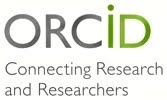The image features the text "ORCID" prominently displayed in a large font. The letters 'O', 'R', and 'C' are in a bold, gray color, while the letters 'I' and 'D' are in the same large font size but colored in an olive green. The 'I' has a distinct dot at the top, maintaining the same size as the other letters, and the 'D' is a regular capital letter. Beneath "ORCID," in a smaller font approximately two-thirds the size of the main text, are the words "Connecting Research and Researchers." Each word starts with a capital letter: 'C' in Connecting, 'R' in Research, and 'R' in Researchers, while the word "and" is in lowercase. The phrase "Connecting Research and Researchers" is in a consistent gray color. The overall design balances the contrasting colors of gray and olive green to emphasize "ORCID" while clearly presenting the tagline below.